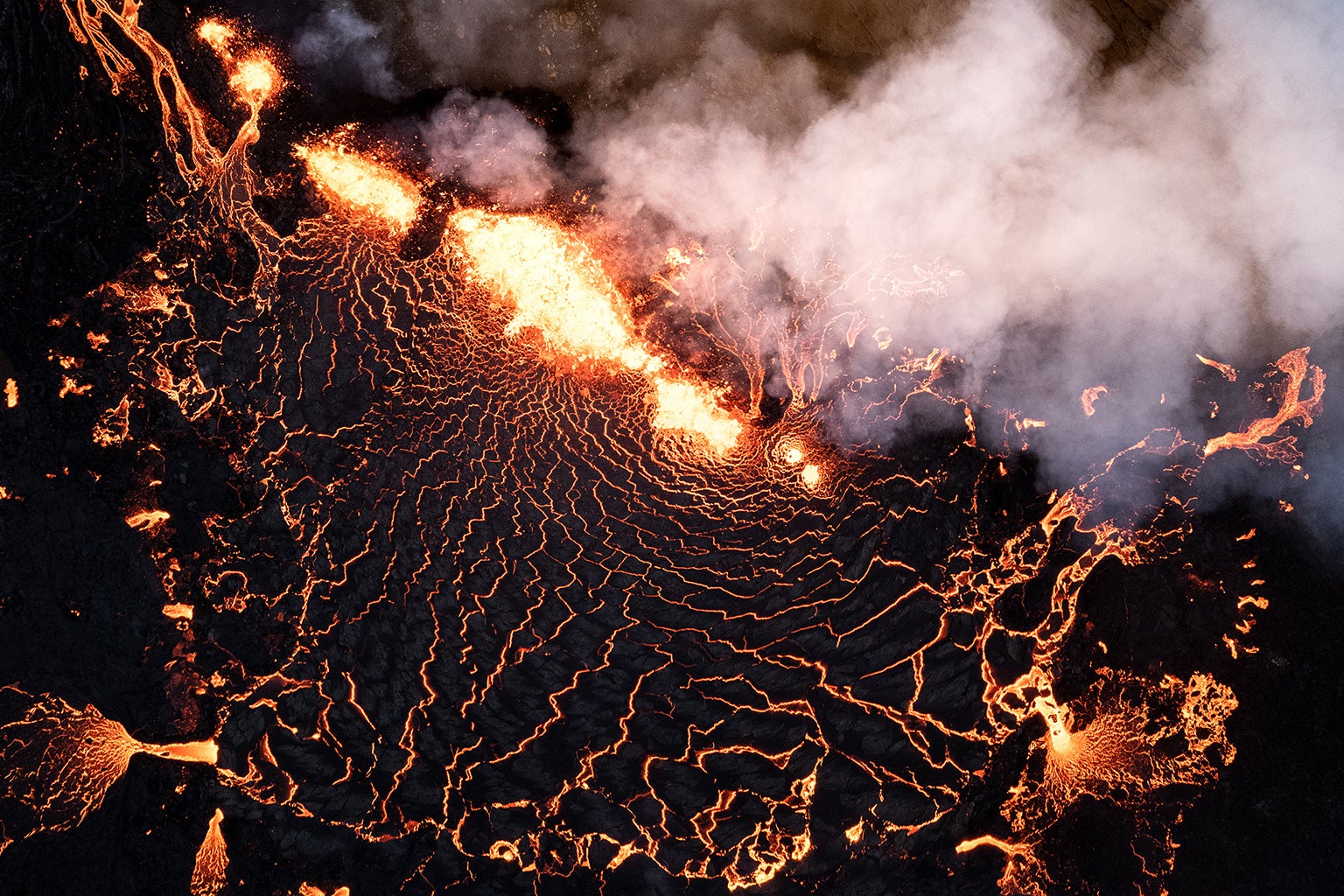The image captures an aerial view of a volcanic eruption in vivid detail. At the top right corner, thick gray smoke billows upward, shrouding part of the frame. Below this smoky veil, luminous orange and bright yellow lava emanates from the volcanic crater. The molten lava flows downward, creating a striking contrast against the dark, almost blackened rock surface. Jagged and branching lines of bright orange magma snake through the rugged, black terrain, resembling the complex network of a nervous system. These brilliant strands of hot magma highlight the dynamic motion of the lava as it courses through the surrounding landscape, setting the stage with a fiery interplay of colors and textures. The overall scene dramatically showcases the raw and powerful beauty of nature's molten fury.